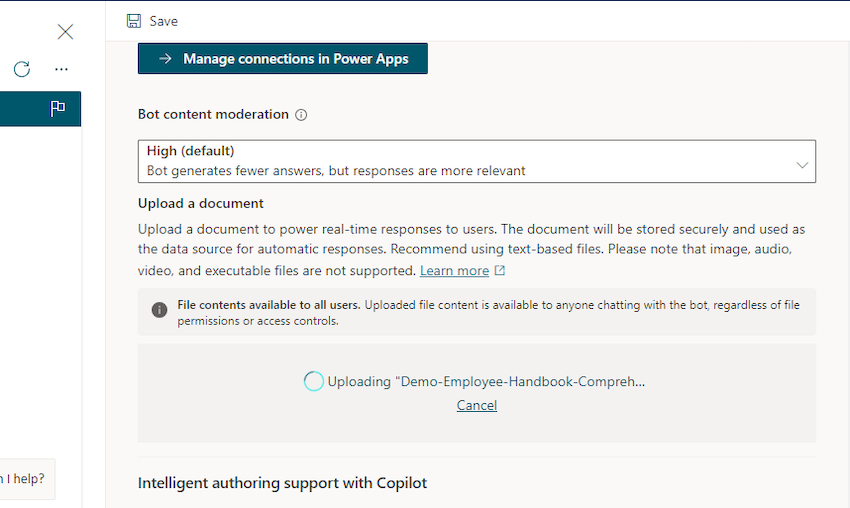Certainly! Here's a cleaned-up and detailed caption for the described image:

---

The image features an interface on a white background. At the top, there is a save icon depicted by a floppy disk logo, accompanied by the word "Save" in dark blue or black font. Below it, a dark blue clickable box with white text and a white arrow reads "Manage connections and Power Apps." 

Further down, there is a section labeled "Bot content moderation" with an information icon next to it, represented by a lowercase 'i' encircled within a black circle. This section includes a description stating, "High (default): Bot generates fewer answers but responses are more relevant," indicating that more information can be accessed by clicking.

Beneath this, there is a prompt to "Upload a document," followed by explanatory text related to the document upload process. 

At the bottom, there are two light blue informational boxes. The first box, situated on the left with an information icon (lowercase 'i' encircled), states in black text: "File content is available to all users. Uploaded file content is accessible to anyone chatting with the bot regardless of file permissions or access control."

The larger, second light blue box features a loading symbol, which is three-quarters full in a light blue shade, and reads, "Uploading demo employee handbook comprehension." This suggests that a document upload is currently in progress. 

Finally, across the bottom of the interface, black text states "Intelligent authoring support with Copilot," indicating the use of the Copilot AI tool within this interface.

---

This caption provides a comprehensive description of the image while maintaining clarity and attention to detail.